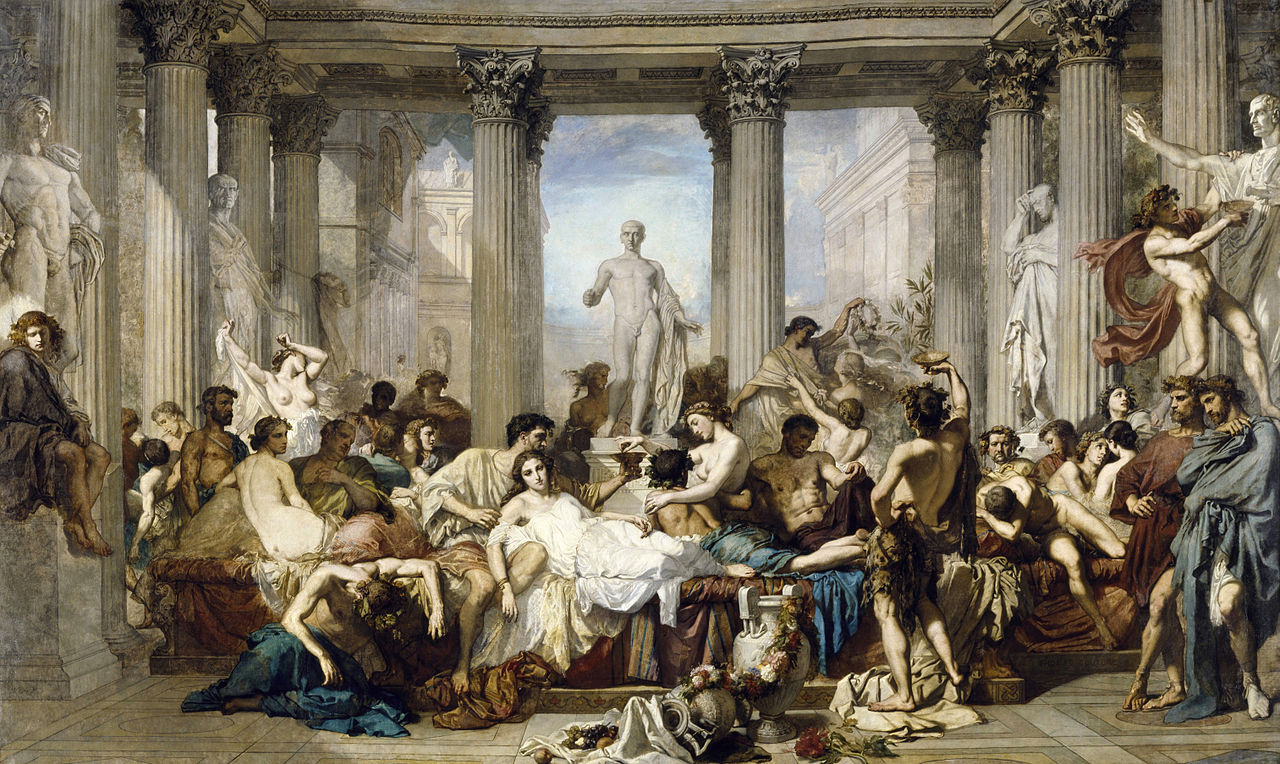The painting likely depicts a scene from ancient Greek or Roman times, featuring a grand, opulent palace with tall, white pillars dominating the architecture. Scattered throughout the scene are several statues, reminiscent of renowned classical sculptures such as Michelangelo's David. In total, there are five to six statues placed throughout the space. 

The room is filled with numerous individuals in varying states of leisure and attire, some wearing colorful robes akin to togas, while others are partially or fully unclothed. The somewhat chaotic arrangement of people suggests a scene resembling a lavish party aftermath, with men and women lounging, standing, sitting, and interacting with one another in various poses, some with limbs draped casually, others in more intimate, suggestive positions.

Additionally, the scene includes various objects strewn around, such as vases and remnants of food, further emphasizing the revelry that likely occurred. The backdrop features a view of the sky and distant buildings, hinting that the setting might be in a central, significant location within a town. Overall, the painting evokes a sense of indulgence and relaxation, characteristic of a grand Roman or Greek social event.